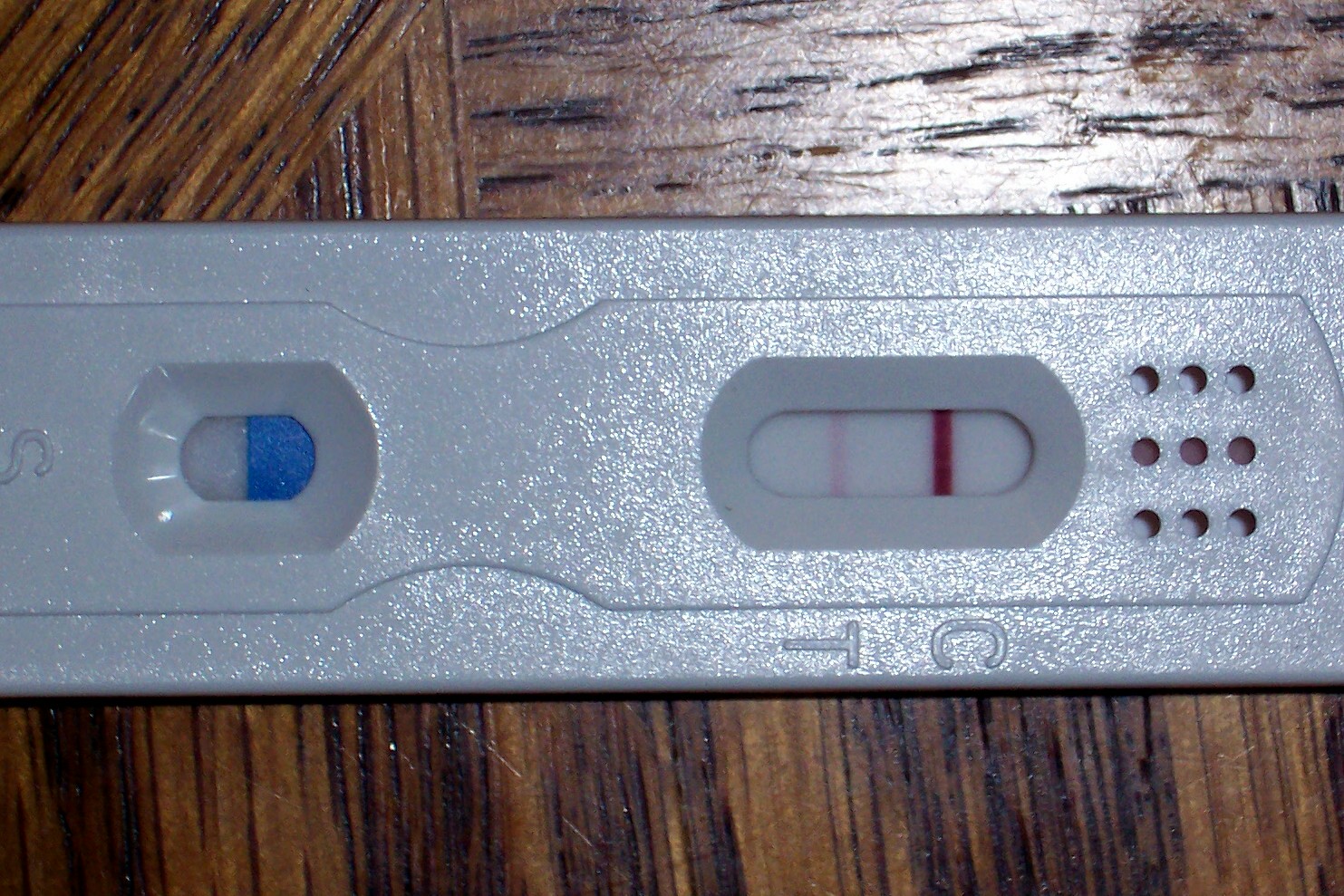The image features a wooden tabletop as the background, prominently displaying a pregnancy test at the center, oriented horizontally. The pregnancy test device is primarily gray and has a distinctive rectangular shape with inward curving sides, giving it a silhouette reminiscent of a band-aid. 

In the lower section of the test, there are indented labels, "C" and "T," molded into the plastic. The central part of the test contains an oval window, which is internally divided into two parts: the left side is white, while the right side is blue. Adjacent to this, on the right side of the device, another oval window is present. This second window features a white segment to the left, and a gray segment to the right, displaying a faint red line on the left and a darker red line on the right.

Further to the right of the oval windows, there are three small, evenly spaced circular holes arranged in a trio, adding to the detailed structure of the pregnancy test.